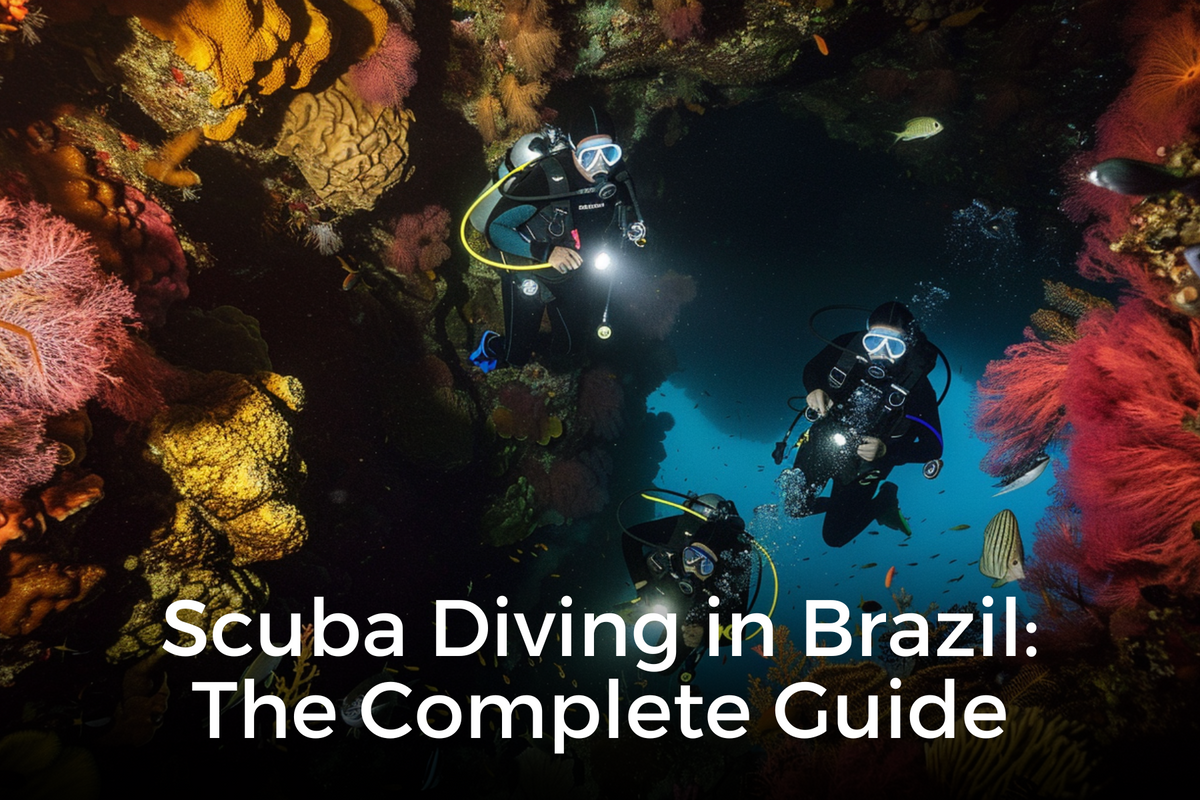The photograph depicts three scuba divers fully equipped with blue goggles, diving deep into the ocean surrounded by a diverse marine environment. The text at the bottom of the image reads "Scuba Diving in Brazil: The Complete Guide," suggesting the image might serve as a title page for a presentation or guidebook. Among the colorful, though somewhat muted, aquascape, a range of lush textures and colors of coral—reds, yellows, pinks, greens—can be observed. The coral varies from feathery to hard and rough in appearance, providing a vibrant backdrop. Larger fish swim around the scuba divers, while a school of smaller fish is visible in the darker blue depths of the background. Despite the overall dim light of the deep ocean, the divers use flashlights to illuminate their surroundings, highlighting the vivid corals and fish.